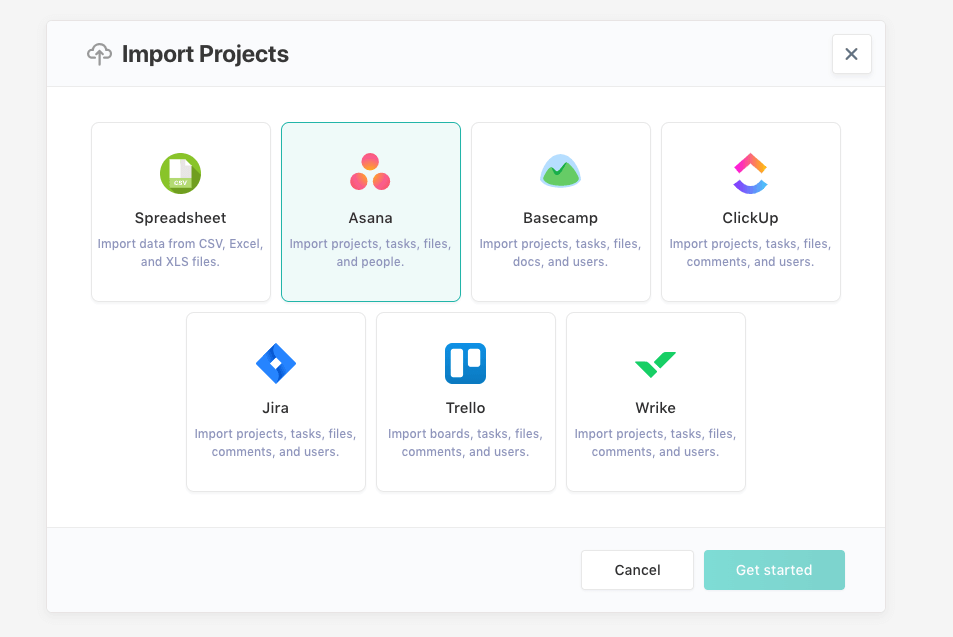This is a detailed description of the provided image:

The image is a cropped screenshot of a web page, revealing only a portion of the entire layout. The background of the webpage is an extremely light gray. Within this background, there is a central rectangular section with a pure white background, which is just slightly wider than it is tall. 

At the top left corner of this white rectangle, bold black text reads "Import projects." Directly beneath this heading, there are four distinct import options presented in a single row:

1. **Spreadsheet**: Represented by a small green icon symbolizing a spreadsheet. The accompanying text states, "Import data from CSV, Excel, and Excel S files."
2. **Asana**: Presented within a small blue square featuring a light blue background. The Asana logo, consisting of three red dots arranged in a triangular formation, accompanies this option.
3. **Basecamp**: Displayed with its logo, which resembles a dome with a mountain inside it.
4. **QuickUp**: Identified by a logo that looks like an upturned line representing a smile, with a small pyramid shape above it.

Below this row, another row features three additional options:

1. **Jira**: Listed as an import option.
2. **Trello**: Included in the import choices.
3. **Wrike**: Noted as "Reiki" but spelled "W-R-I-K-E" in the image.

The arrangement and visual icons provide a clear and structured way to select different project import methods.